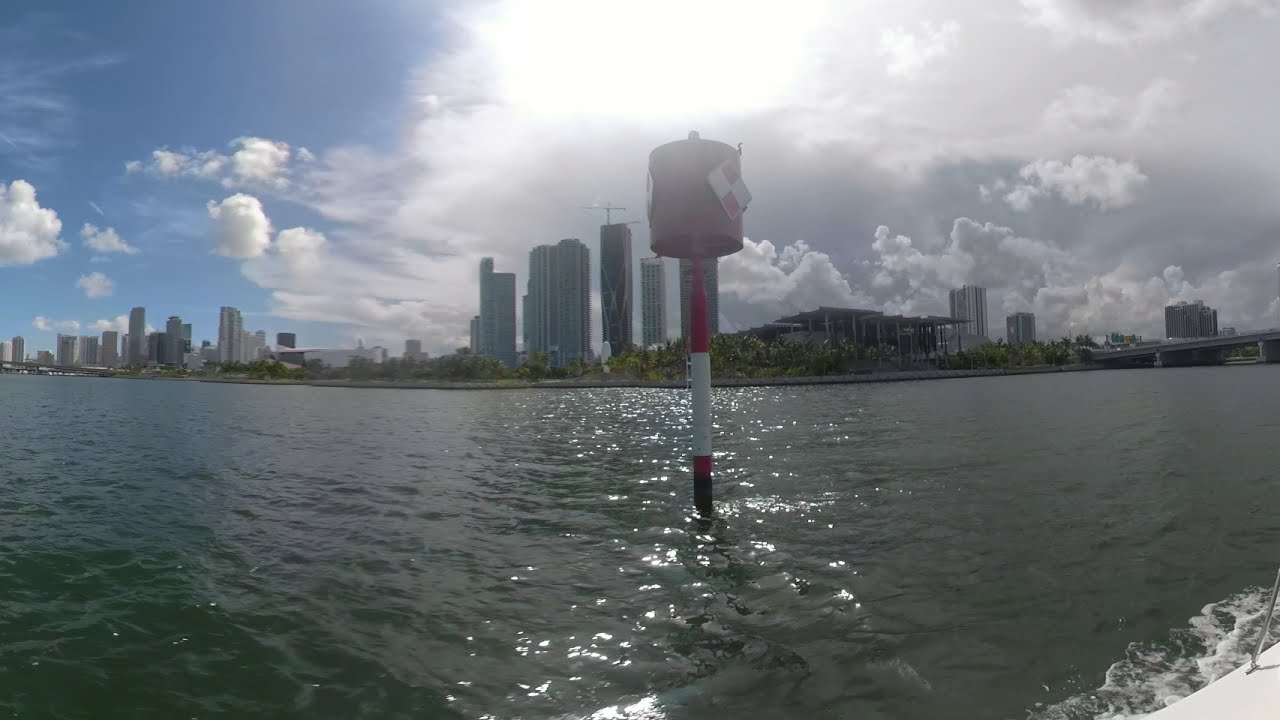The photograph, taken outdoors during the daytime, captures a panoramic view of a large city surrounded by a wide waterway. The sky above is a mix of a bright blue horizon on the left and large, fluffy gray and white clouds on the right, with a bright white sun partially obscured but shining through the center. The skyline is dotted with tall skyscrapers, indicative of a bustling urban environment. Across the waterway, two bridges can be seen: a road bridge on the far left and another bridge on the far right. In the foreground, the water is rippling and reflects the sunlight in various sections. Rising six to eight feet out of the greenish water is a prominent red-and-white striped pole topped with a red cylinder and a checkered flag, likely a weather buoy equipped with instruments. This detailed scene illustrates a serene yet dynamic interaction between urban development and natural waterways.